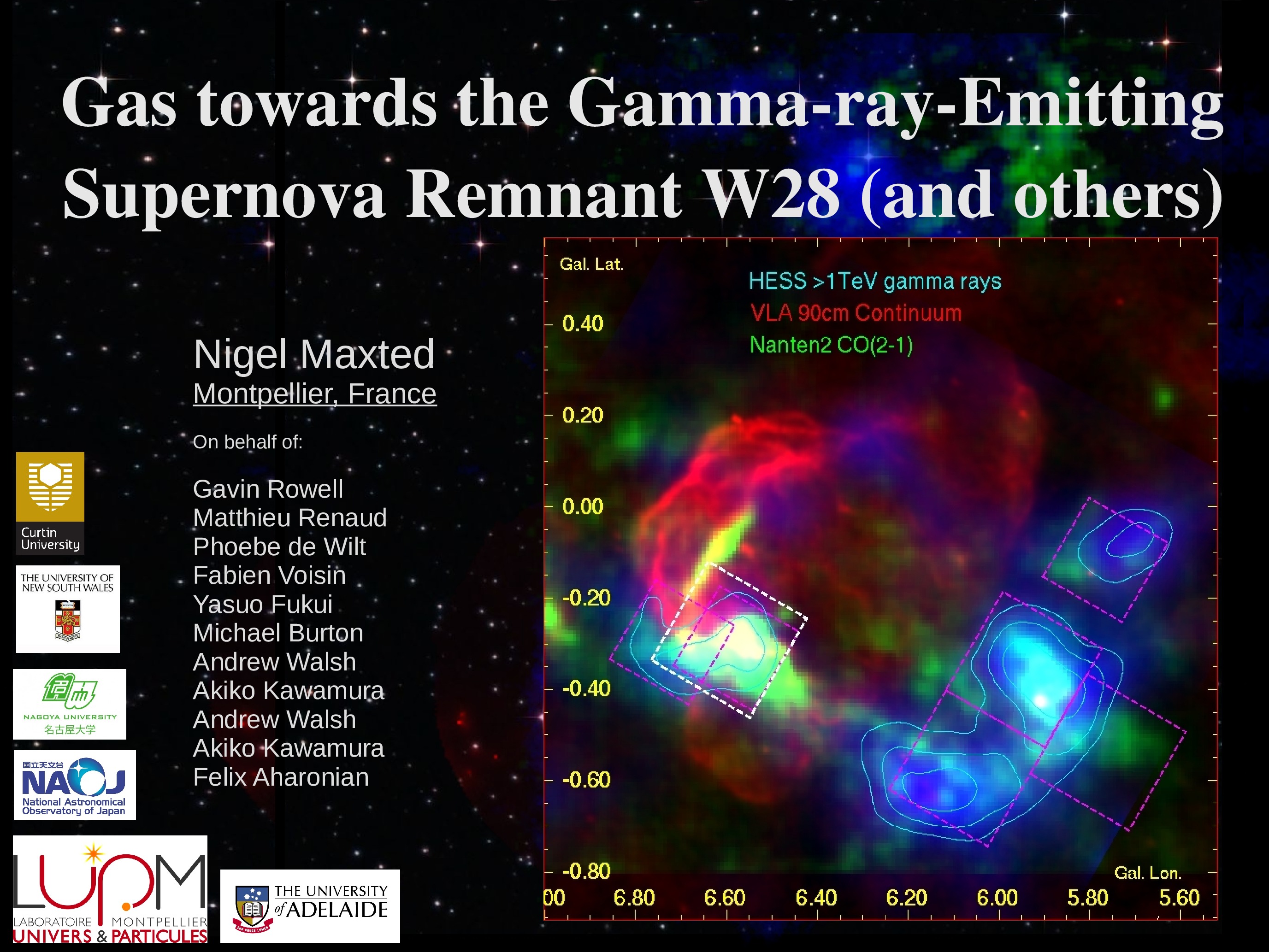The image is an informational poster designed with a striking black background that mimics the night sky, scattered with stars to create a galactic feel. Its prominent title in white font reads "Gas Towards the Gamma Ray Emitting Supernova Remnant W28 and Others." Below the title, the text in smaller white font lists contributors: Nigel Max Ted, Matt Peel, your France, on behalf of Gavin Rowell, Matthew Renaud, Phoebe DeWitt, Fabian Voisin, Yasso Fukui, Michael Burton, Andrew Walsh, Akio Kawamura, and Felix Aharonen.

On the left-hand side, the poster features names like the University of Adelaide, with several badges including institutions such as Krillin University and University of Suramese. A detailed graph occupies the right-hand side, showcasing bright shades of red, green, and blue to illustrate different data sets. Labels in blue, red, and green represent different types of data: "HESS-TV Gamma Rays," "VLA 90cm Continuum," and "NANTEN 2 CO(2-1)" respectively. The graph contains a scale that spans vertically from -60 to 40 and horizontally from 0 to 560, aimed at capturing the gamma ray spectrum of the supernova remnant W28.